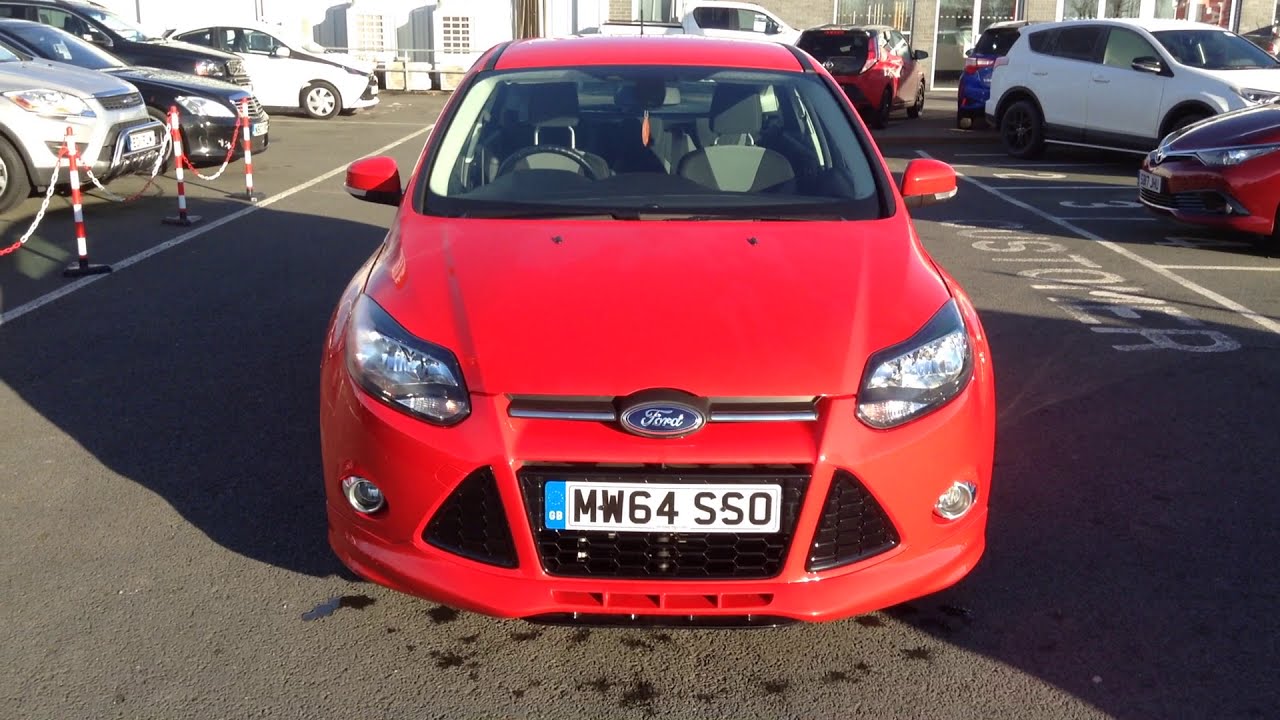In this detailed outdoor image, likely taken in the middle of the day at a car dealership or parking lot, the focal point is a red Ford car positioned directly in the center of the frame. The car is viewed head-on, displaying a prominent navy blue Ford logo with cursive silver lettering on the grille. The scene is bustling with various vehicles. To the left of the red Ford, four cars, including a damaged vehicle and a red and white striped parking blockade, are neatly parked. To the right, another four to five cars are visible. Directly behind the red Ford is a white pickup truck. The parking lot is marked with white lines indicating parking spaces, and the ground is made of asphalt, resembling a typical road. The red Ford car features a foreign license plate that reads MW64SSO, characterized by a white background, black characters, and a blue vertical stripe on the far left. Various other vehicles in the lot include a white van, a red sedan, a red minivan, a white sedan, a black car, and a black truck. The vehicle interiors and trunks are somewhat discernible, although no drivers are present in the image. The scene captures a mix of colors including gray, white, black, red, blue, light blue, tan, and a hint of yellow.